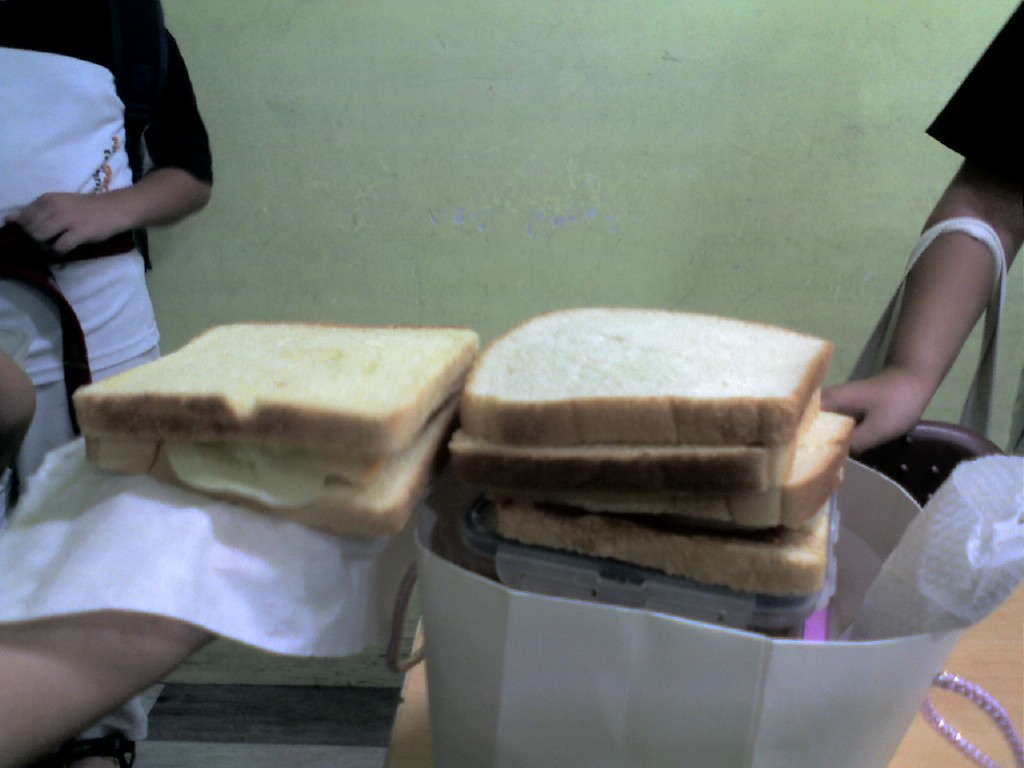This digital indoor photograph features two individuals flanking the edges of the frame against a creamish yellow-green wall background. On the left, a person wearing a white shirt with black elbow-length sleeves, along with a visible black sash, is seen. On the right, another person dressed in a black short-sleeved shirt has a strap over their arm, likely carrying a bag. 

The central focus is on the food and items in the foreground. An upturned hand on the left side is seen holding a napkin with a sandwich made of two pieces of white bread, possibly with a cheese filling. Adjacent to this, a white shopping bag featuring lavender-pink handles contains several unwrapped slices of white bread with a golden tan crust. Stacked near the top of this bag are more pieces of bread, forming what appears to be another sandwich. Various items, including boxes, are visible inside the bag, contributing to a somewhat cluttered scene.